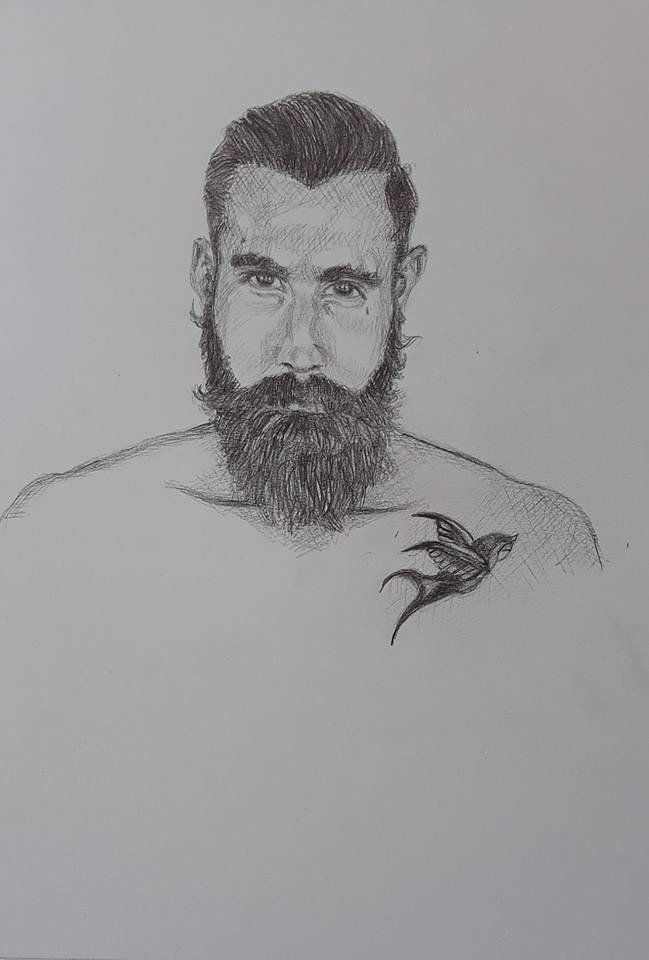This detailed pencil sketch portrays a man from the upper shoulders to the head. He has broad shoulders, accentuated by a prominent tattoo of a swallow on his left pectoral. The swallow's face is angled upward toward the top-right corner of the image, while its wings and tail drape diagonally downward toward the bottom-left. The man's facial features are distinctly marked by a very thick beard and mustache, completely obscuring his mouth. His bushy eyebrows frame a long, tall, rectangular face. He has long, flowing brown hair, and all these elements come together in an intricate pencil rendering, highlighting the artist's attention to detail in texture and expression.